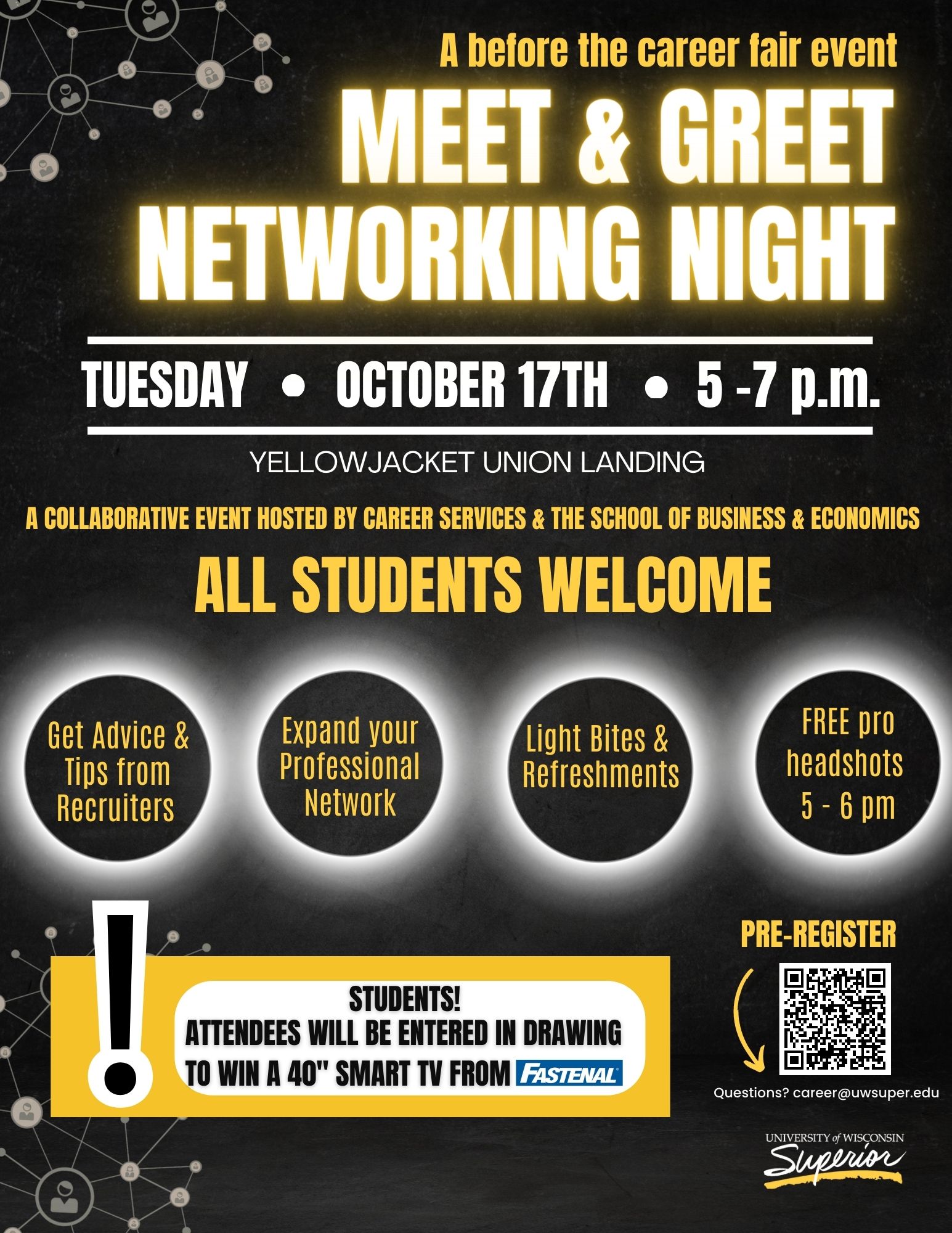The poster, set against a black background, advertises a "Meet and Greet Networking Night" event, intended as a precursor to a career fair. Dominating the top left is a graphic of interconnected nodes, symbolizing networking, with people connecting to lock icons. To the right in bold orange or yellow text, it reads "Meet and Greet Networking Night." The event, open to all students, will be held on Tuesday, October 17th from 5 to 7 PM at the Yellow Jacket Union Landing. Highlights of the event include opportunities to get advice and tips from recruiters, expand your professional network, enjoy light bites and refreshments, and benefit from free professional headshots offered between 5 and 6 PM. Additionally, student attendees will have the chance to enter a drawing to win a 40-inch smart TV from Fastenal. A QR code for registration is positioned at the bottom right, adjacent to another networking graphic similar to the one at the top. The event is a collaborative effort hosted by Career Services and the School of Business and Economics.